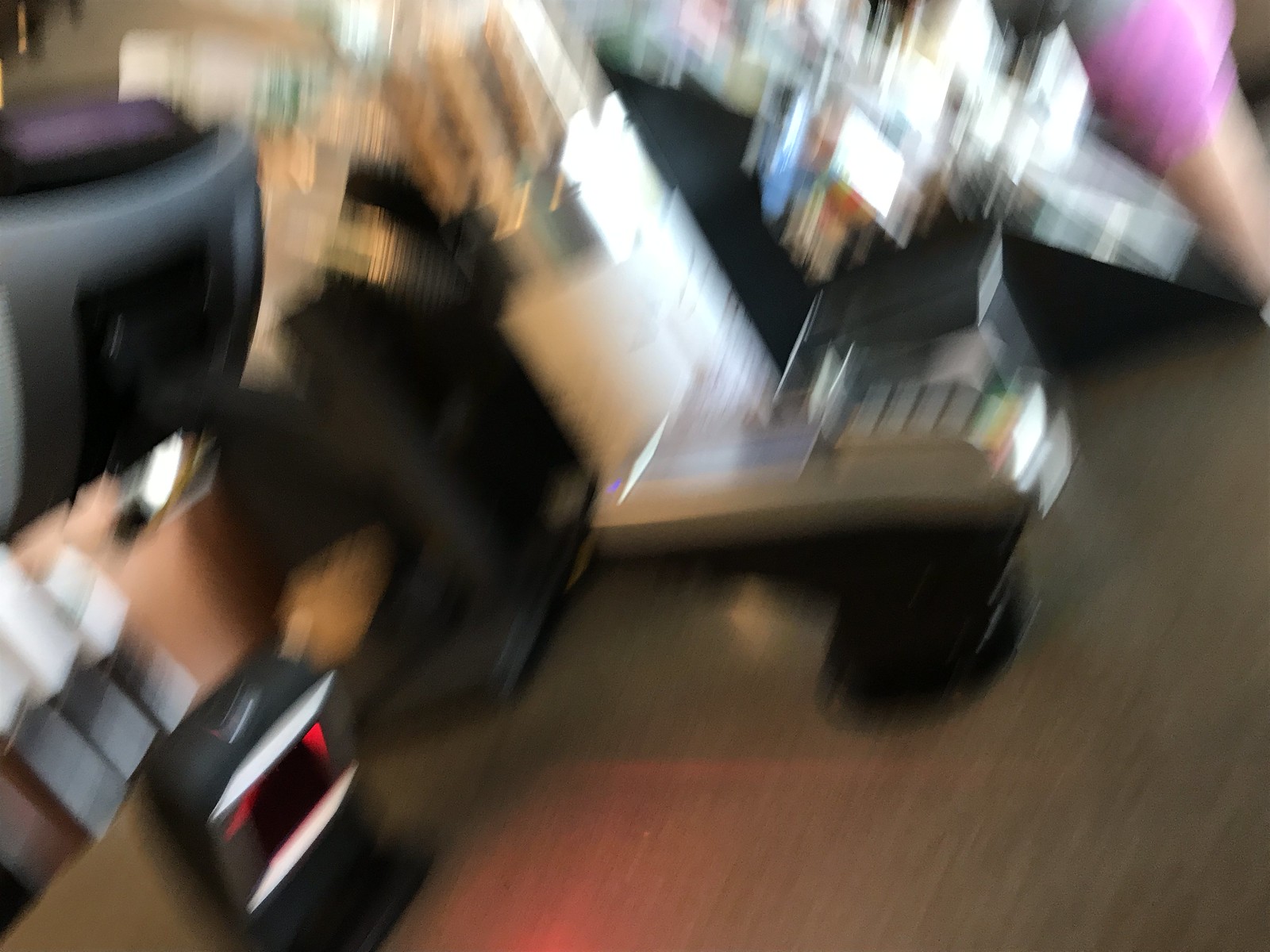The image depicts a cash register checkout machine, possibly located at a Circle K gas station or a similar convenience store. The image is quite blurry, but several key features can be discerned. Visible components include an EBT card reader and a Visa card reader, offering multiple payment options for customers. There is also a barcode scanner for processing various products. Although the image is too indistinct to identify all the elements clearly, the setup appears typical for a retail environment, designed to facilitate quick and efficient transactions for a myriad of items.